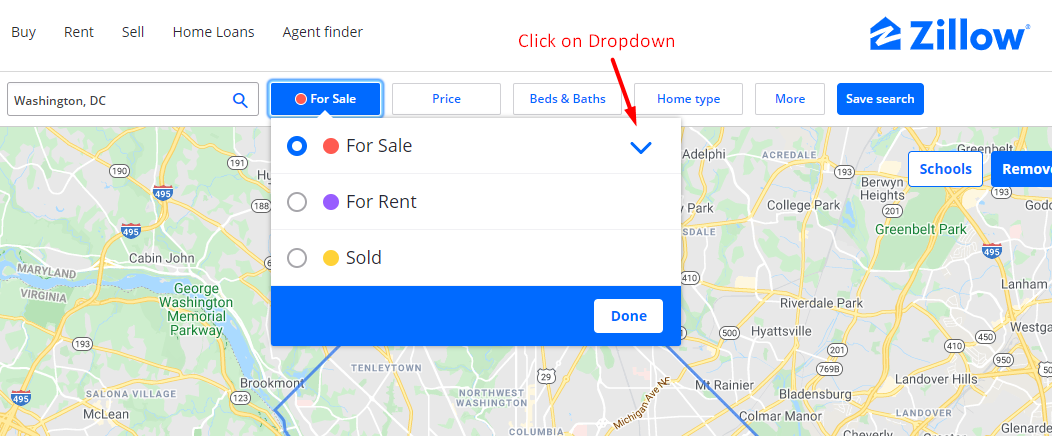In this screenshot of a web page, we see Zillow’s company name and logo positioned in the upper-right corner. The logo features a blue house with a white "Z" inside, and the name "Zillow" in blue text appears to the right of the logo. The main content is a detailed map rendered in light green, gray, yellow, and blue hues. 

The map highlights several geographical features and locations. On the left side, it shows parts of Maryland and Virginia, including the city of McLean, Virginia, which is situated in the lower-left section. In Maryland, Cabin John is noted along with the George Washington Memorial Parkway. Interstate 495, a major north-south route, is also visible in Maryland.

On the right side of the map, we see Greenbelt Park, depicted as a greened-out area. Further south, the map identifies the cities of Hyattsville, Landover Hills, and Lanham. The color-coded map provides a clear and comprehensive view of these regions and their connections.